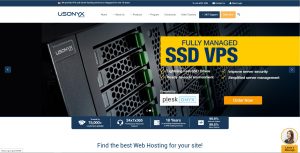The image depicts a webpage displayed in an extremely zoomed-out view. The layout begins with a top section featuring a black background. Directly below, the background shifts to white, where several categories are aligned in very small text. Positioned to the right are two rectangular icons: one black and the other orange.

Below this header section, there is a sizable image set against a black background, appearing to show part of a tire. Displayed prominently in this area are the words "fully managed SSD VPS," along with some smaller white text beneath it. Adjacent to the text are two rectangular buttons, one white and one orange.

Further down, a black rectangle contains four selectable options. At the very bottom of the page, there is a statement beginning with "find the best web hosting for your," but the final word is too small to decipher. This section concludes with a white background, and in the bottom right-hand corner, there is a stamp-like design with an orange rectangle, completing the image.